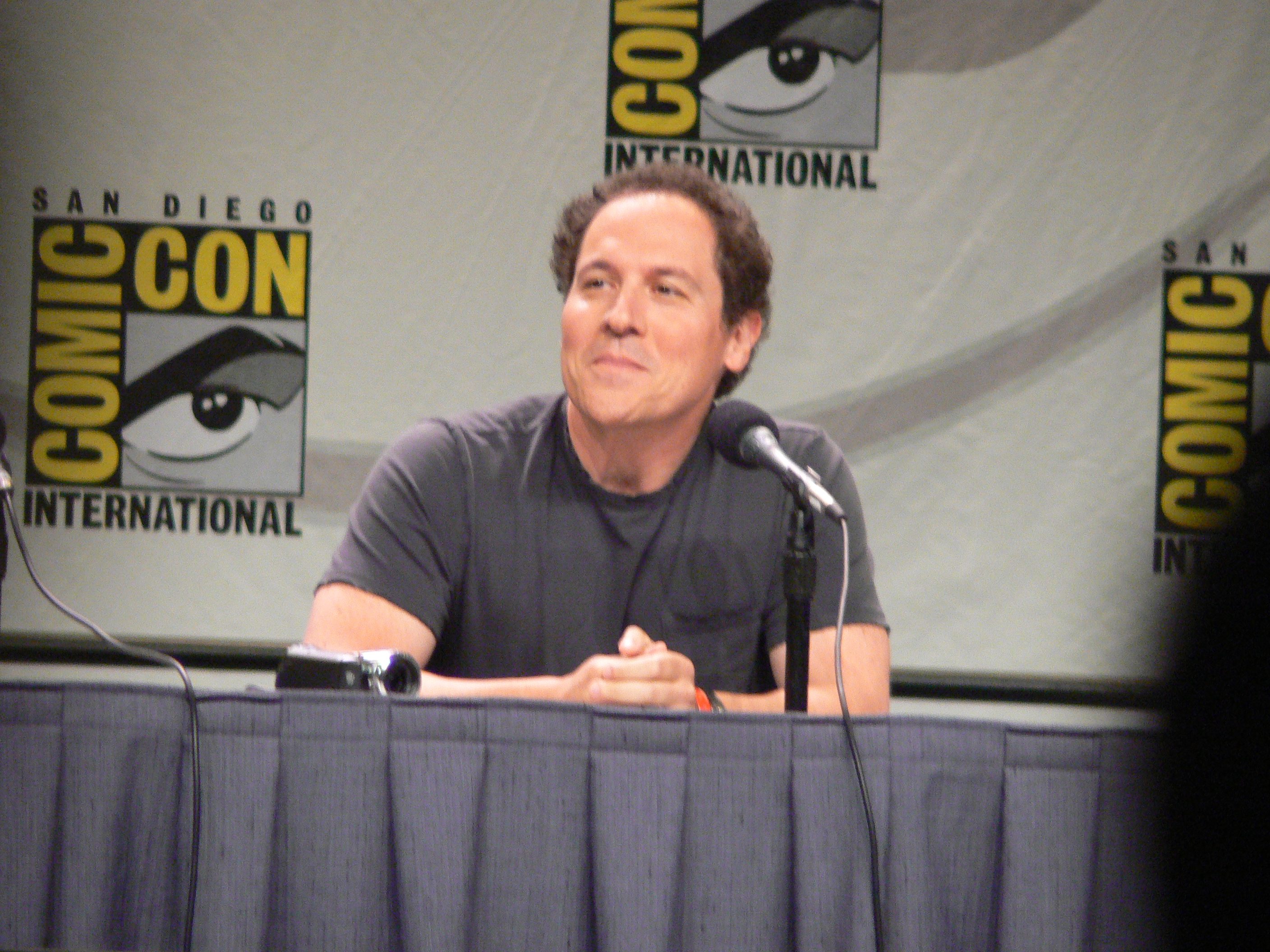The image features actor Jon Favreau seated at a table during Comic-Con in San Diego. He is captured leaning on his elbows with his hands clasped in front of him, speaking into a black microphone mounted on a stand. The table has a gray cloth covering. Favreau, with his short, curly brown hair, smirks as he appears to be listening to a question. He is wearing a gray short-sleeved t-shirt and a wristband on his left wrist. The backdrop consists of a white banner repeated with the San Diego Comic-Con International logo, which includes the text "San Diego" in black, "Comic-Con" in yellow, and an eye symbol in a square frame. A shadowy figure can be seen on the far right of the image, contributing to the bustling atmosphere of the event.